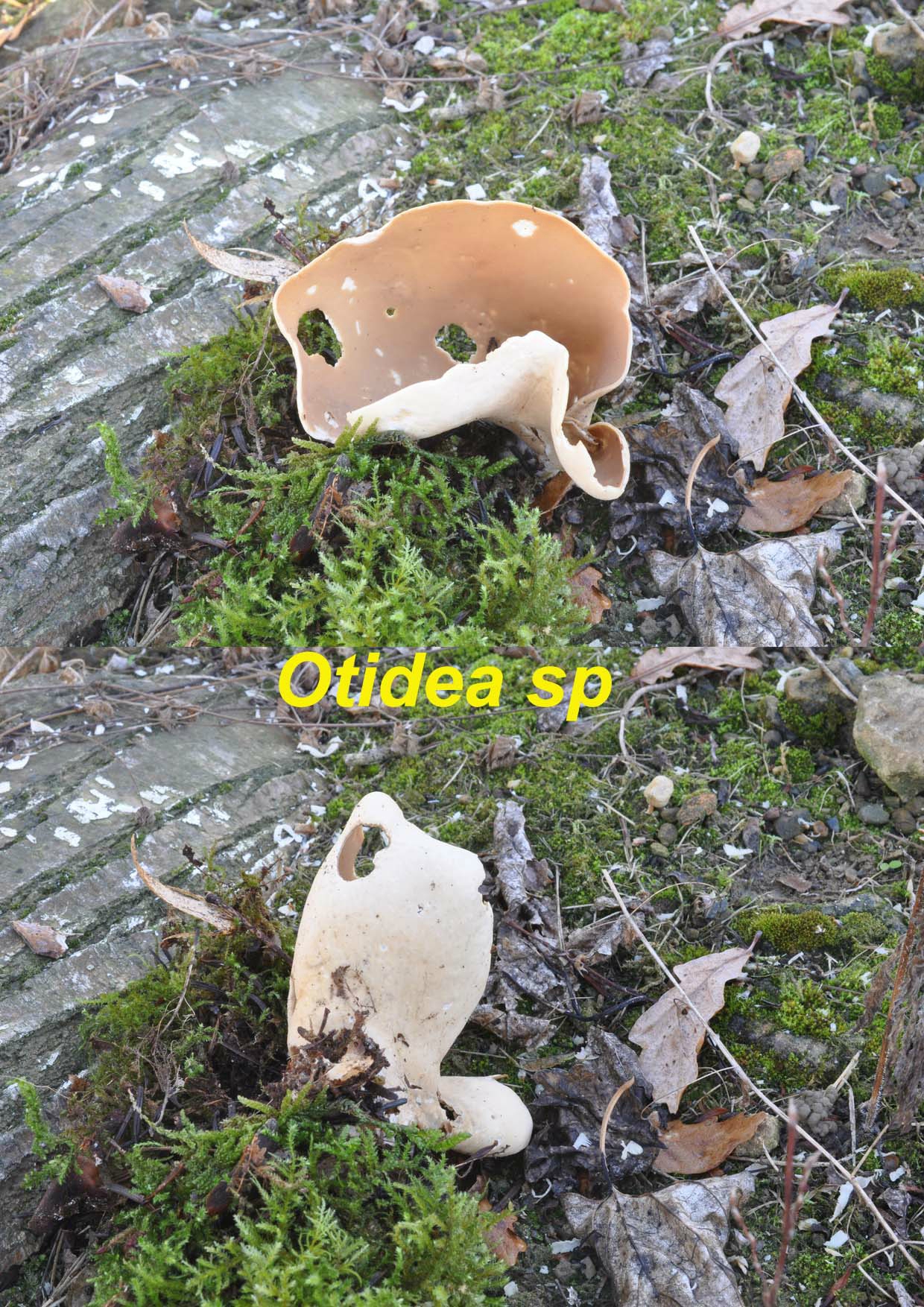In this outdoor photograph, the scene features a mix of earthy elements, including dirt, grass, weeds, and various plants. Strewn across the ground are several broken, flexible plastic pieces with numerous holes, some appearing to be in an L-shape or 7-shape, showing both their inside and outside surfaces; the plastic appears tan on the outside and light brownish-tan on the inside. Surrounding these pieces are dead brown leaves, twigs, and patches of straggly moss. The ground also has some gray and white rocks, some with rectangular shapes and diagonal lines, with vines emerging from them and moss or mildew growing in the crevices. The predominantly natural scene, which suggests a fall or winter setting due to the presence of dying leaves, is further contextualized by the caption "Otidia SP" displayed in yellow text in the center of the image.